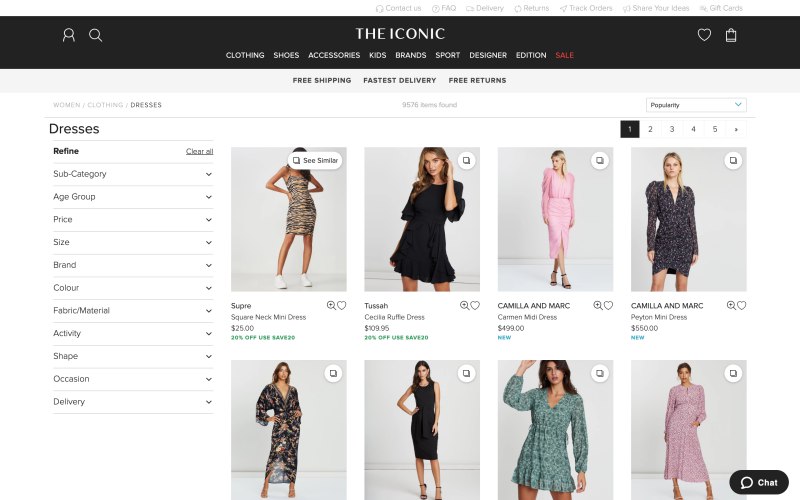The screenshot depicts a desktop view of the homepage of The Iconic website. The topmost bar features a white background with gray icons and text for various customer services such as contact support (represented by a headset), FAQs (a question mark), delivery information (a truck), returns (two circling arrows), order tracking (a paper airplane), sharing feedback (a megaphone), and gift cards (a magic wand).

Directly below, a black navigation bar is present showcasing a generic profile icon for account access, a magnifying glass for searches, and "THE ICONIC" in bold white text. This bar also includes a heart icon for favorited items and a shopping bag for cart contents.

The following section features a white text menu with categories including Clothing, Shoes, Accessories, Kids, Brands, Sport, Designer, Edition, and Sale—the latter highlighted in red text. Beneath this menu, another white bar promotes key services with black text: "Free Shipping," "Fastest Delivery," and "Free Returns."

The on-screen user is navigating the Women's Clothing and Dresses section. Filtering options include subcategory, age group, price, size, brand, color, fabric/material, activity, shape, occasion, and delivery, all accessible via expandable dropdown menus. A notable count of 9,576 items is displayed as available. Additional sorting options include popularity filters.

Visible on the screen are products from this category displayed in a grid format, showcasing eight dresses, four per row. Features such as zooming into the product image, adding items to favorites, and price range filters (from $25 to $550) are available. The displayed dresses vary in style and color, including pink, black, green, multicolor floral, and tiger stripes, with lengths ranging from above-the-knee to below-the-knee.